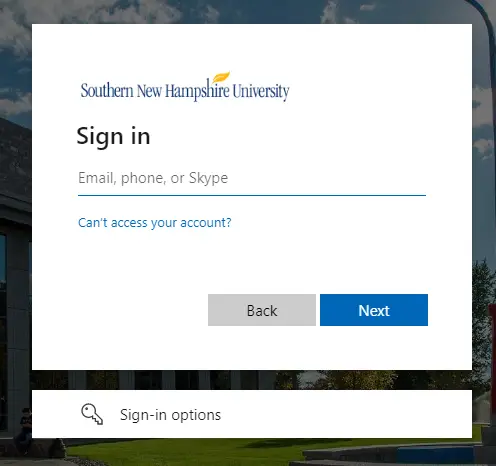This image is a login page for Southern New Hampshire University's website. The page includes options to sign in using email, phone, or Skype, highlighted by a blue line indicating the selected method. A blue link labeled "Can't access your account?" followed by a question mark provides help for those having trouble logging in. The "Back" button is gray, allowing users to navigate to a previous page, while the "Next" button is blue, guiding users to the next step in the sign-in process. Below these buttons, a small key logo appears, indicating additional sign-in options.

The background image on the login page features a scenic view of the university campus. The sky is a vibrant blue with scattered white clouds. To the right, part of a pole is visible amid lush green grass and shaded seating areas. Trees enhance the natural beauty of the scene, and the university buildings stand prominently in the background, contributing to the overall picturesque setting.